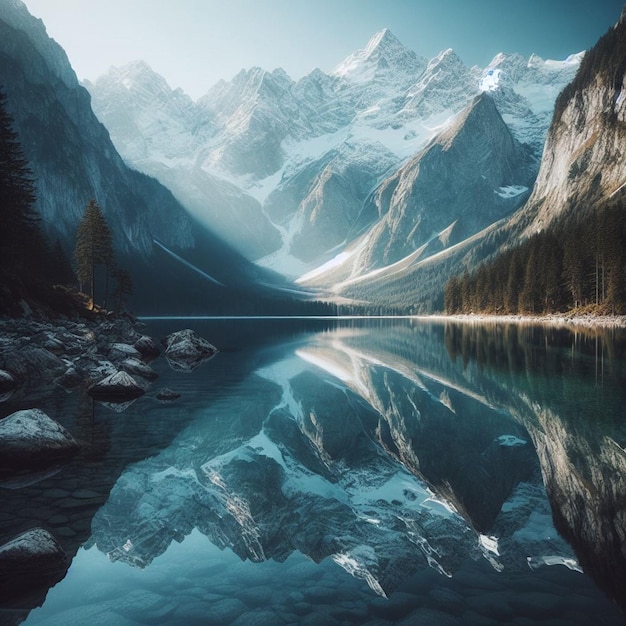This captivating image depicts a serene mountain lake nestled in a valley, surrounded by snow-covered mountains. The water, a stunning shade of blue, mirrors the majestic peaks, creating the illusion that the mountains are both above and below. The clarity of the water reveals stones and boulders submerged just a few feet deep, particularly concentrated towards the left side. On either side of the lake, the steep mountains rise sharply, adorned with layers of snow. Tall, dark green pine trees line the shores, especially prominent on the left, where they contrast with several large gray boulders. The tranquil, reflective surface of the lake captures the pristine beauty of the snowy mountain landscape, making it appear as if the entire scene is doubled in the still water.